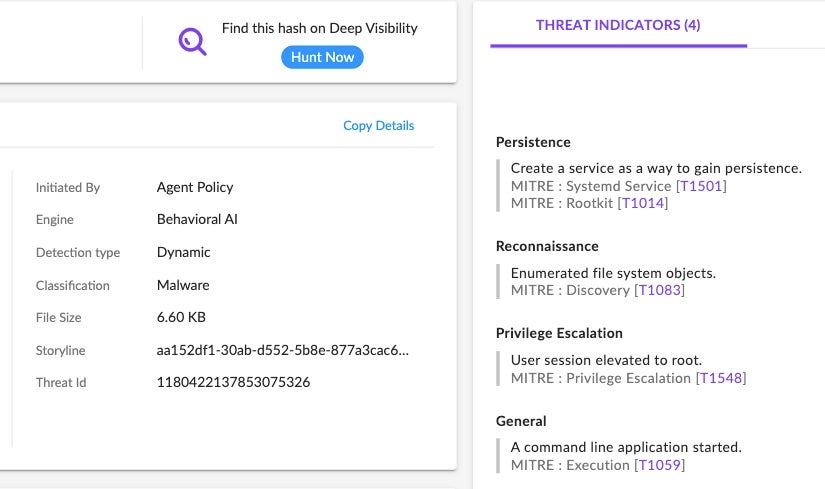This image is a detailed screenshot of a cybersecurity application interface designed for threat analysis. On the left side, the screenshot displays a section titled "Find this hash on Deep Visibility," prompting users to conduct a search. The search indicates it was initiated by the Agent Policy Engine via Behavioral AI, with the direction type classified as Dynamic and the threat type as Malware. The file size is noted as 6.60. A storyline identifier is present, represented by a string of letters and numbers, followed by a field labeled "Threat ID," which also contains a unique numeric string.

On the right side, the image showcases a section named "Threat Indicators," which is divided into four categories:

1. **Persistence**: This category indicates that the threat attempts to maintain a foothold by creating a service.
2. **Reconnaissance**: It highlights that the threat performs activities such as enumerating file system objects to gather information.
3. **Privilege Escalation**: This signifies that the threat evaluates user sessions to escalate privileges to the root user.
4. **General**: It notes that a command line application was started, likely part of the threat's execution.

Overall, the screenshot is comprehensive, emphasizing detailed threat behavior and indicators to aid in cybersecurity analysis.